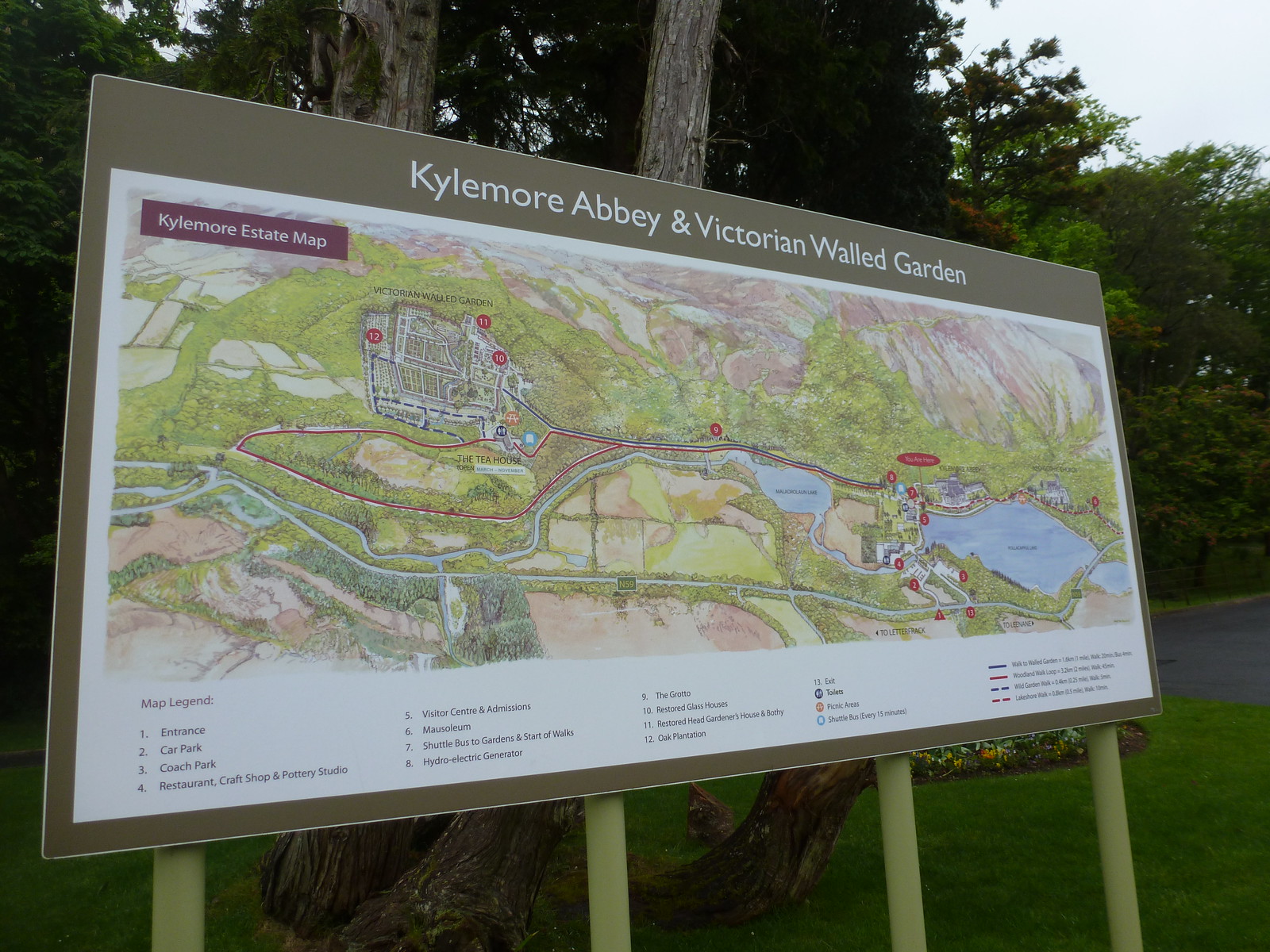The image is a colorful outdoor shot featuring a large rectangular map mounted on four yellow poles. The map prominently displays "Kylemore Abbey and Victorian Walled Garden" in white text against a gray background, with a thicker gray border at the top. The top left corner identifies it as the "Kylemore Estate Map." Central to the graphic is a detailed drawing of the abbey, garden, and surrounding areas, with points of interest marked by red-circled numbers. Below the map, a legend lists these points: 1 is the entrance and car park, 3 is the coach park, 4 indicates the restaurant, craft shop, and pottery studio, and 5 marks the visitor center and admissions. Other key locations include the mausoleum (6), shuttle bus to gardens and walks (7), hydroelectric generator (8), along with additional points somewhat out of focus. The map also explains routes, distances, and amenities like restrooms and picnic areas.

In the backdrop, there are several tall, deciduous trees with hints of orange, suggesting the onset of fall. The well-maintained grass patch is visible on the bottom right, along with a slightly obscured circular flower garden featuring yellow and white flowers. Behind the sign, the image shows a verdant landscape with a mix of grassy areas and what appears to be a blacktop courtyard or parking lot.